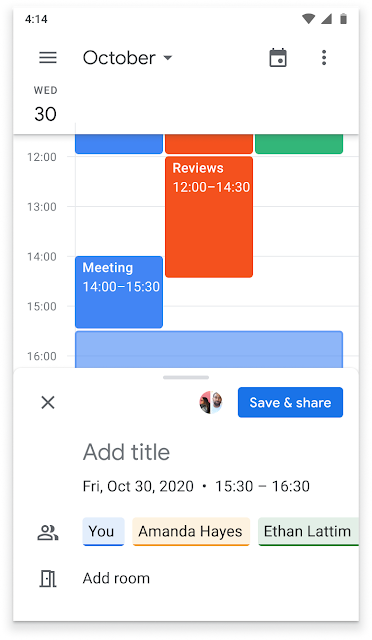The image is a screenshot of the Google Calendar app captured on a mobile device. At the top left, the time "4:14" is displayed, alongside symbols indicating Wi-Fi connectivity, cellular signal strength, and battery life on the top right. The app is set to display events for Wednesday, October 30th. The interface features a clean white background with black or dark gray text.

Time slots are organized into color-coded blocks, primarily using blue, red, and green, representing different events and timespans on the calendar. Each block corresponds to specific hours of the day, such as 12:00 to 14:30 and 14:00 to 15:30.

A pop-up window dominates the lower part of the screen, featuring options to save and share the calendar event. The pop-up includes an X button on the left to close it and the account owner's avatar on the right. The event is titled "Friday, October 30th, 2020, 15:30 to 16:30" and lists participants: You, Amanda Hayes, and Ethan Lattin. There's also an option to add a room, suggesting the function might be used for scheduling classes or meetings. The layout is straightforward and user-friendly, designed for efficient scheduling and planning.